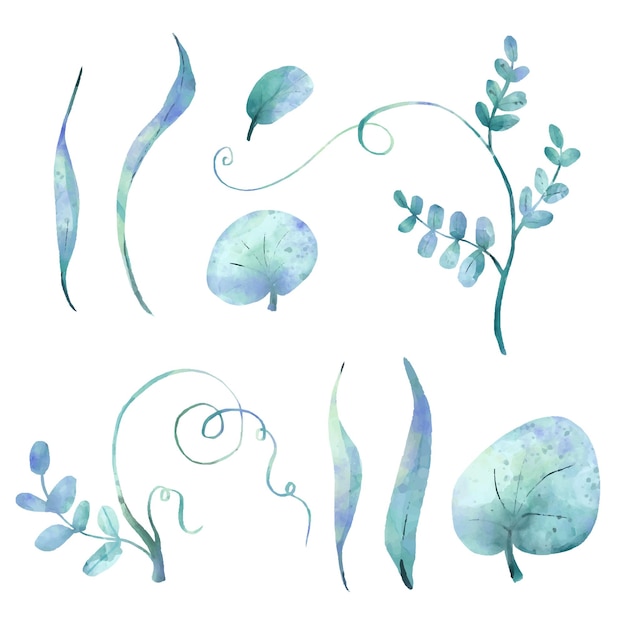The image is a simple yet elegant design featuring various plant leaves arranged against a pristine white background. The drawings are rendered in harmonious shades of blue and purple, lending a watercolor-like quality to the graphic. The leaves are showcased in different styles and sizes, illustrating a diverse array of plant shapes. In two rows, the top row contains five elements: two thin, willowy leaves on the left, followed by two lily-style leaves, and concluding with a plant that has a curvy stem adorned with sub-stems and leaves. The bottom row mirrors this arrangement with a curvy stem on the left, followed by willowy leaves, and ending with a lily on the right. This meticulously crafted graphic not only celebrates the diversity of plant forms but also highlights the beauty of subtle variations in leaf structure through its cohesive color scheme and detailed design.